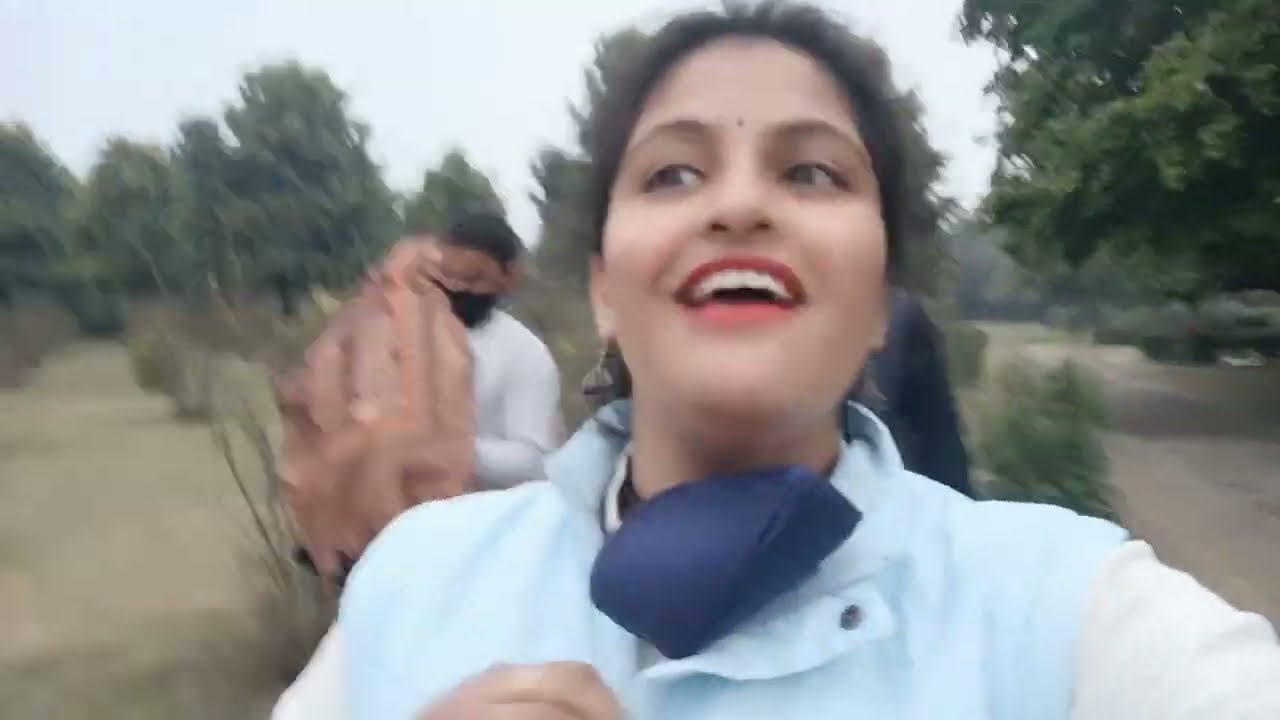In this blurred outdoor photo, a woman with black hair and a bindi between her eyebrows is captured in mid-movement as she smiles, revealing a row of teeth. She has on red lipstick, dangly earrings, and a white shirt underneath a light blue jacket or vest. A blue surgical mask hangs around her neck. Her right arm is outstretched beyond the frame, and part of her left hand is visible as she looks off to the left in apparent joy. The background features a bright blue sky, scattered with trees, hinting at a serene forest-like setting, possibly in autumn or spring given the brown ground. Standing behind her is a black man in a white shirt and brown cab, with a dark mask covering his face, carrying a large brown leather item, possibly a saddle, over his shoulder. The image exudes a sense of exultation and togetherness amidst a natural, tree-filled landscape.